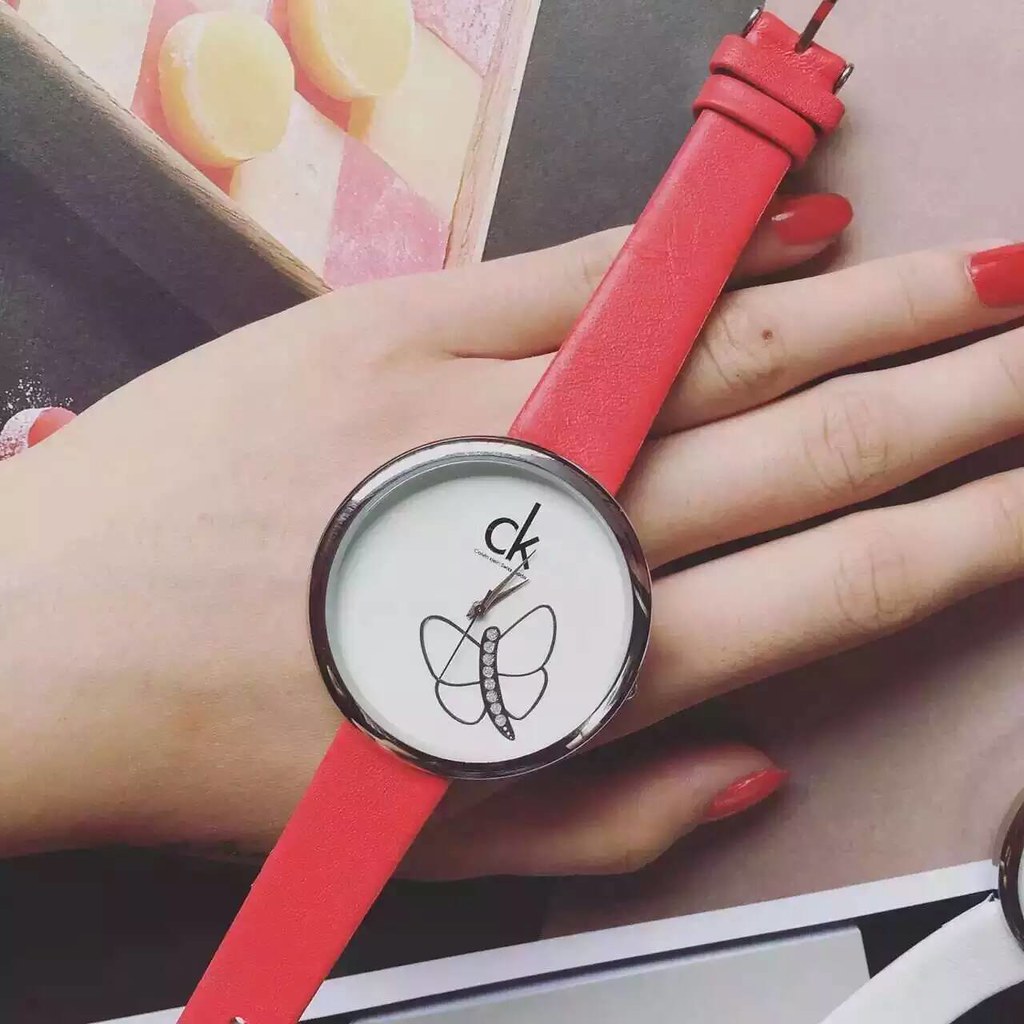This photograph showcases an exquisitely elegant watch with a minimalist design. The watch face is pristine white, adorned solely by a delicately outlined butterfly motif, seemingly encrusted with small diamonds that add a touch of opulence. The absence of conventional hour, minute, and second markers emphasizes its sleek aesthetic, with the only text being the subtle "CK" brand insignia. The watch features meticulously crafted minute, hour, and second hands, set within a refined silver bezel. Complementing the elegance of the watch is a beautiful pinkish-red band, harmoniously matching the fingernails of the woman whose hand serves as the backdrop for this timepiece. In the distant background, a checkerboard is visible, with checkers that resemble intriguing candy pieces, further enhancing the image's unique and captivating composition.